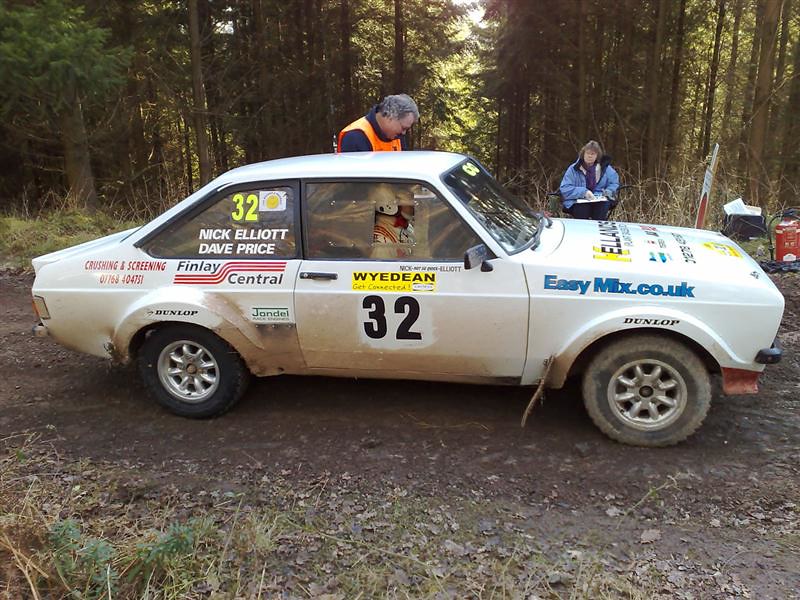The image depicts a classic 1970s-era off-road race car parked on a dirt road in a dense, wooded area. The car, which bears the number 32, has various sponsor decals including Dunlop, easymix.co.uk, Nick Elliott, Dave Price, and Finley Central Crushing and Screening, prominently displayed on its white exterior. The driver's side window appears to be cut out for ventilation. Inside the car, a race driver wearing a white helmet and racing suit is seated. Outside the car, a man in a blue hoodie and bright orange safety vest, with gray hair, stands by the driver's side, looking down at the ground. To the side, a woman with a light blue heavy jacket and a pink scarf sits on a chair, holding a notepad. She is observing the scene, which is illuminated by daylight seeping through a thick stand of pine trees in the background. This setting creates a vivid picture of a race checkpoint or pit stop amidst a forested off-road trail.